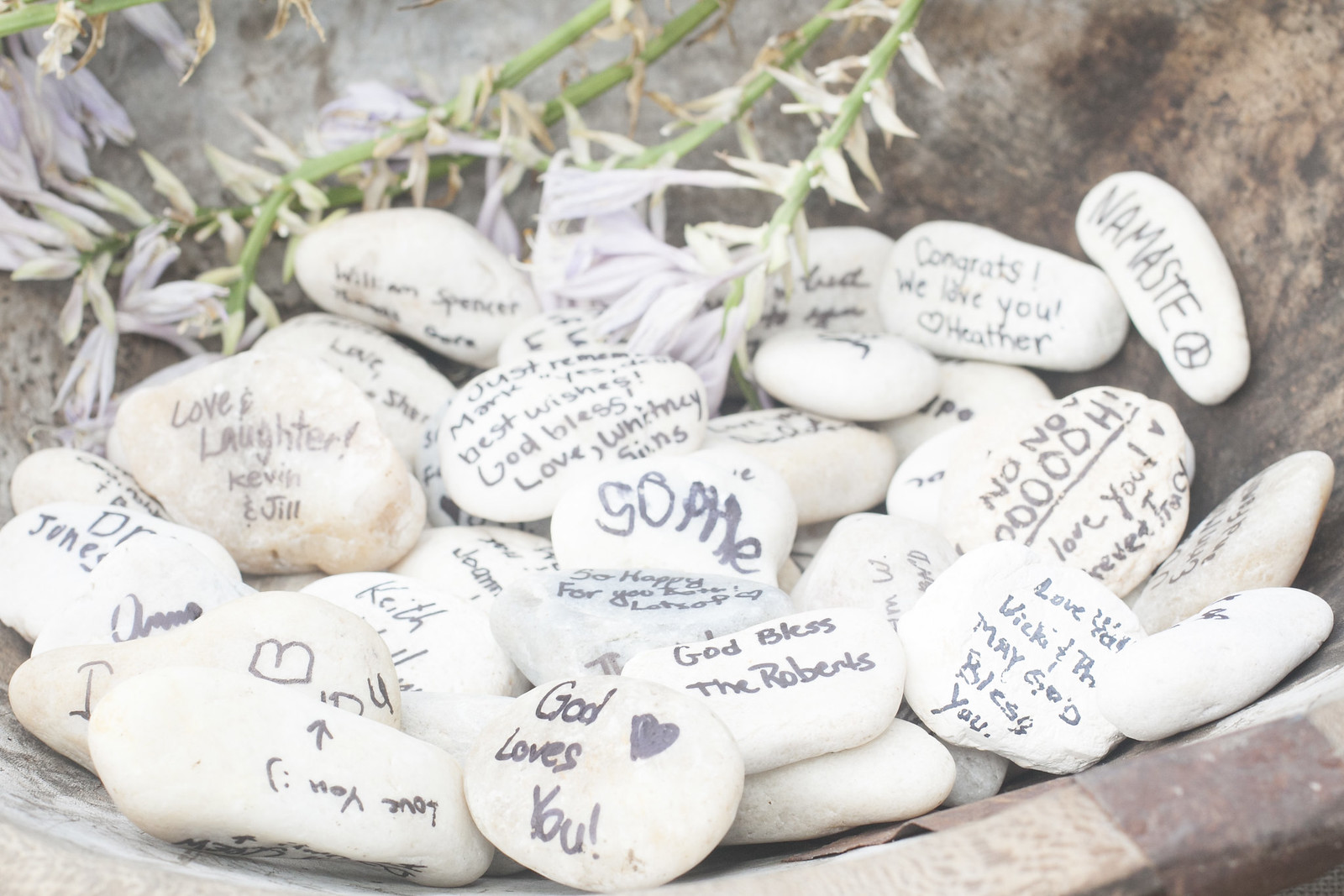In the image, a weathered, multicolored cauldron, displaying hues of white, brown, and black and resembling a stone bowl, is filled with approximately 25 flat, oval-shaped rocks. These pale gray or white stones are inscribed with various heartfelt messages in black ink, expressing love, blessings, and positive affirmations. Some of the prominent inscriptions include "God loves you," "God bless the Roberts," "Namaste" with a peace sign, "Love and laughter, Kevin and Jill," "Love you," "Just remember, Mark," "Best wishes, God bless, love, Whitney Sims," "Congrats we love you, Heather," and "Love you, Vicki." The names and messages appear to convey a sense of care and community. Amongst the rocks are several somewhat wilted flowers with long green stems and light purple petals, adding a tender touch to the arrangement. The collective display seems to be a thoughtful gesture to remind someone that they are cherished and supported.